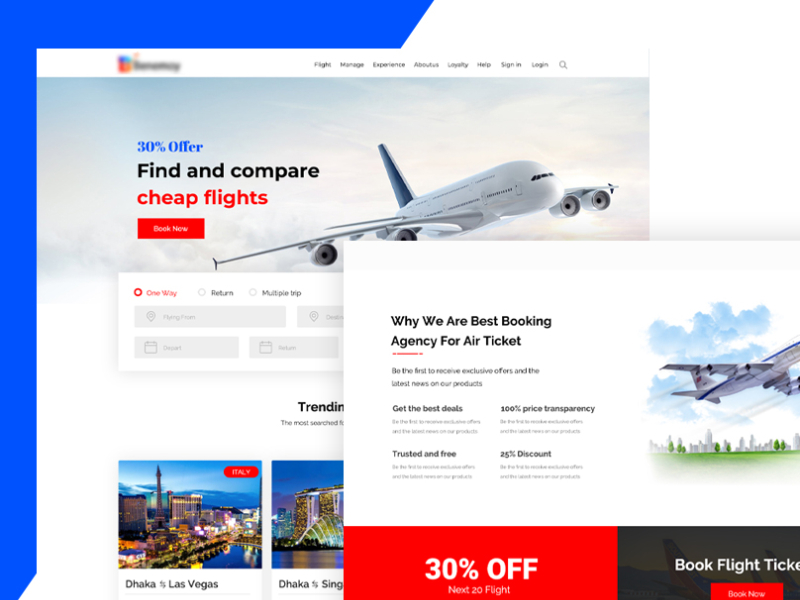The image appears to be a screenshot from a travel booking website, with the company's logo strategically blurred out for confidentiality. The layout has a blue pane on the left side and a white pane on the right. Dominating the visual is an enticing photograph of an airplane soaring among fluffy clouds. Text overlay on the image boldly advertises a "30% Off" promotion alongside a call-to-action: "Find and Compare Cheap Flights. Look Now."

Users are provided with flexible search options: one-way, return, or multi-destination trips. The form fields include the departure location, destination, departure date, and return date. Below these fields, a list of trending routes such as Dhaka to Las Vegas and Dhaka to Singapore is displayed, hinting at popular destinations.

A pop-up window within the screenshot highlights a special offer, claiming, "Wow, we were the best booking agency for air tickets," and offers reasons supporting this claim. The same pop-up emphasizes another compelling offer: "30% off the next 20 flights." Clear calls to action encourage users to "Book Flight Tickets" immediately to take advantage of the deal.